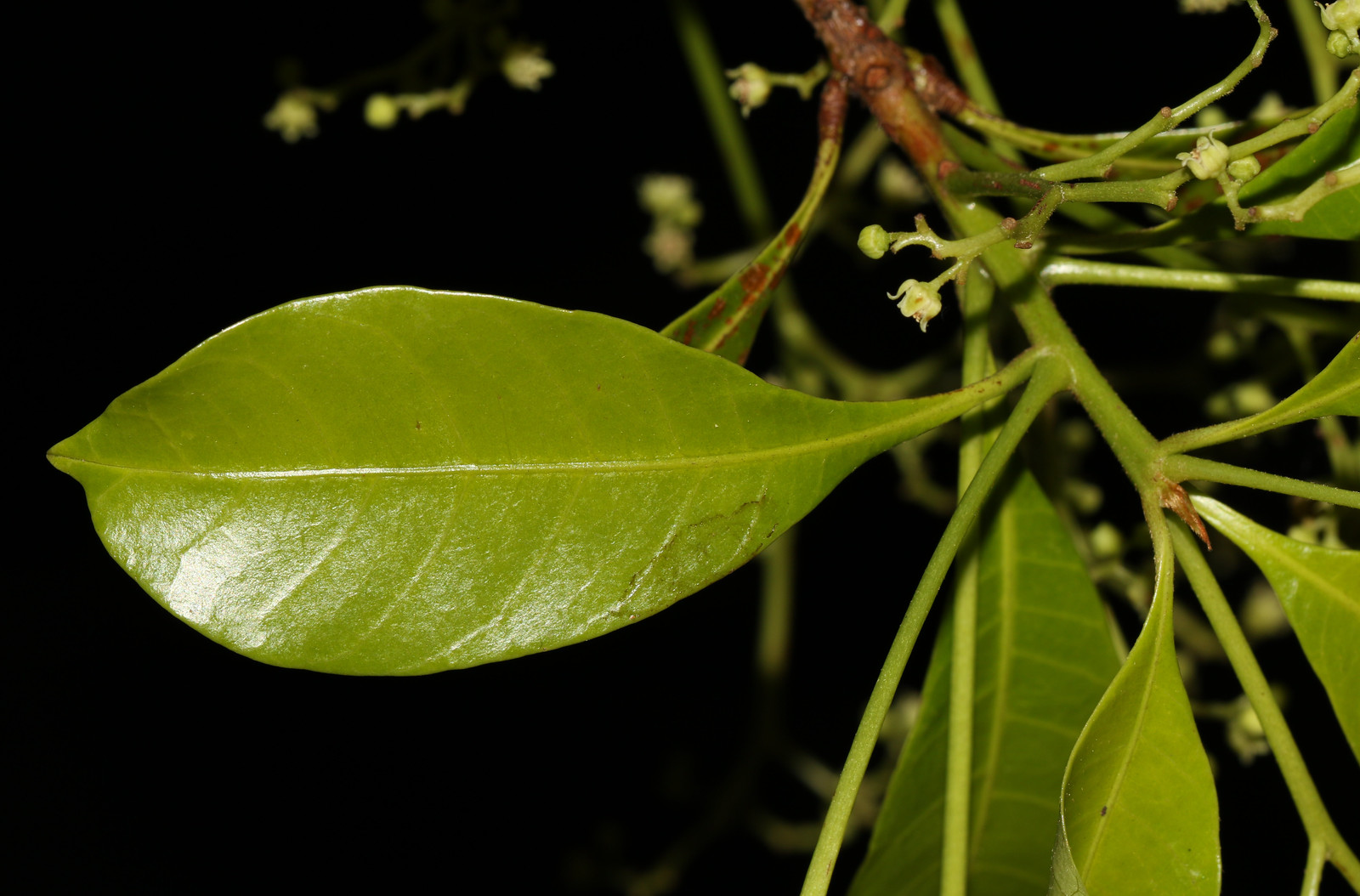The photograph is a close-up, horizontally aligned, rectangular image of a vibrant green leaf prominently displayed against a dark, completely black background, suggesting it might be taken at night. At the center, a main teardrop-shaped leaf extends leftward from a brown stem that transitions to green as it branches off horizontally. This primary leaf, glistening with a healthy sheen and noticeable light reflection likely from a flash, draws the viewer’s attention with its bright green color and intricate light green veins. On the right side of the image, several thinner branches are visible, adorned with smaller, downward-projecting leaves and tiny white buds indicating early stages of blooming. The smaller leaves maintain the same green vibrancy, contributing to the natural, lively essence of the plant captured in this detailed botanical close-up.